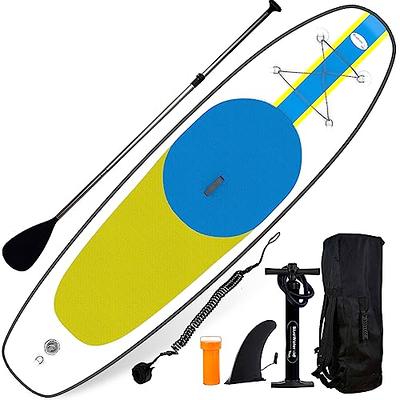The image depicts a computer-generated graphic featuring an inflatable white raft with a blue middle section and a gray top, designed to resemble a kayak. The raft prominently features a blue and yellow circular design complemented by a yellow oval pattern. Positioned next to the raft on the left side is a large paddle with black accents. Scattered on the right side of the image are various pieces of equipment, including a bag, an air pump, a fin, a coiled rope or tube, and a bottle-shaped object. The overall scene is set against a completely white background, evoking a clean and modern aesthetic typical of sports and outdoor gear promotional materials.